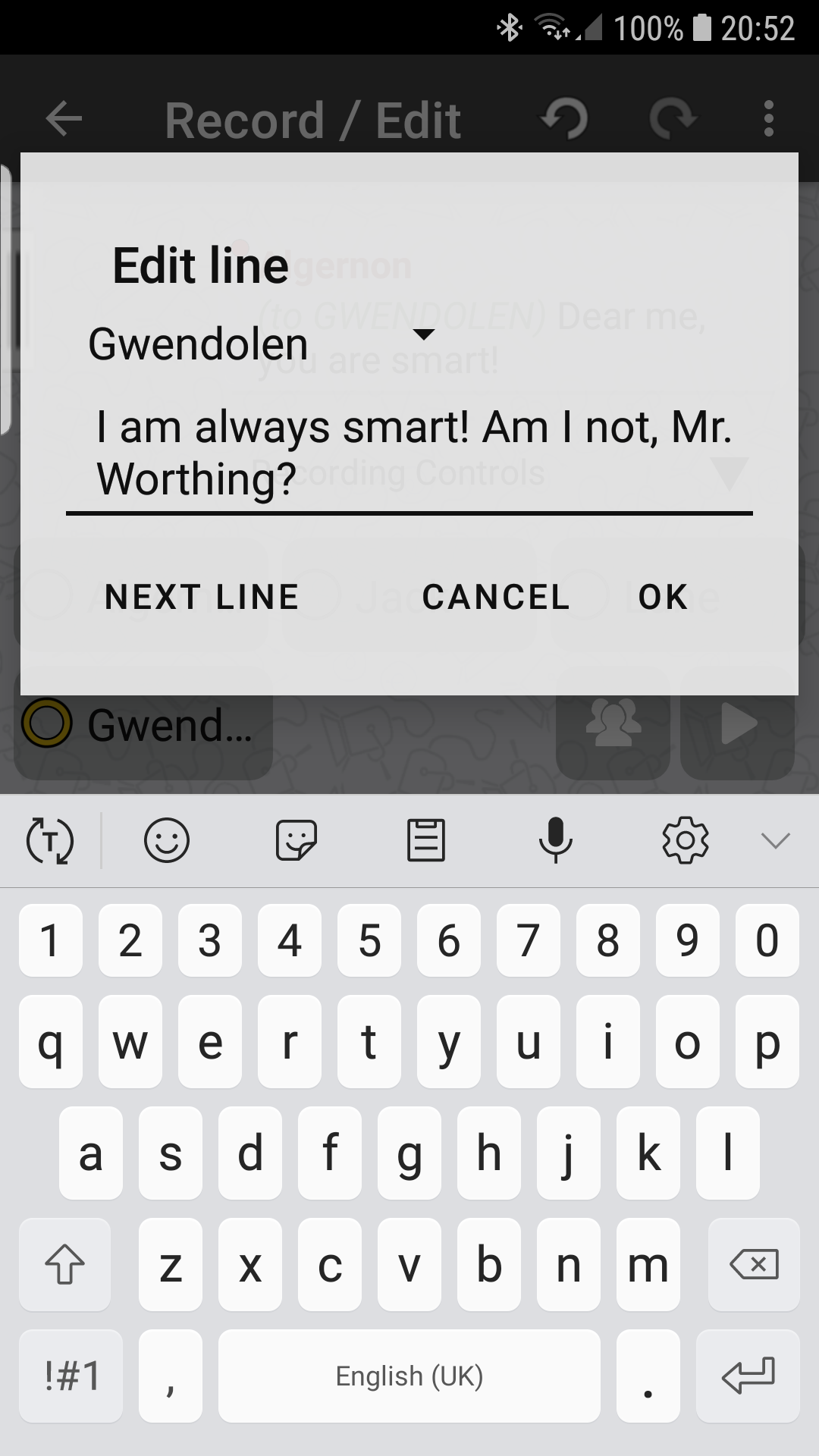The image appears to be a screenshot taken from a smartphone. In the top-right corner, several status icons are visible: a Bluetooth icon, a Wi-Fi icon, a signal strength indicator, a battery percentage reading "100%", a battery icon, and the time displayed as "20:52."

Below the status bar, there is a navigation header with various elements. On the left, there's a back arrow, followed by the text "Record/Edit." Next, are icons for reverse (a circle made out of a line), forward (a clockwise arrow in a circle), and finally, three vertically arranged dots for more options.

The main content of the screenshot is dominated by a large gray text box featuring black text. At the top of this box, it says "Edit line" in bold black text. Underneath, it reads "Gwendolyn" with a downward-pointing arrow next to it. Beneath that, there's black text saying, "I am always smart, am I not Mr. Worthing?" A black underline separates this from the next section, which includes options labeled "Next line," "Cancel," and "Okay." This layout suggests it is part of a text editing or input interface.

Below this text box, an on-screen keyboard with a gray background is depicted. At the top of the keyboard are several icons: a "T" with a circle around it, a smiley face, a square smiley face, a page icon, a microphone icon, a gear (settings) icon, and a downward-pointing arrow. The keyboard includes a number row at the top, followed by three rows of letters. Special function keys flank the left and right sides of the bottom row. The keyboard also displays a space bar, a comma key, and a period key.